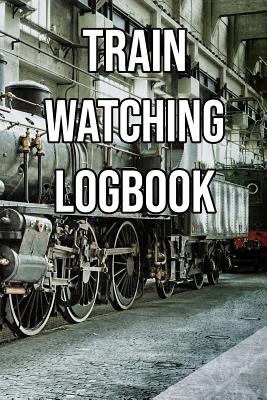The cover of the book prominently features the title "Train Watching Logbook" in a bold, thick white font at the top. The main design dominating the background is an image of a train in motion, moving towards the left side of the frame. The train is depicted passing in front of a building that appears to be constructed from stone, adding a historic or classic architectural element to the scene. The perspective of the image is from a low angle, looking down the side of the train, which allows a detailed view of the left side of the train, particularly emphasizing the wheels and the lower portion of the train cars. The composition captures a sense of movement and the rugged, mechanical beauty of the train.